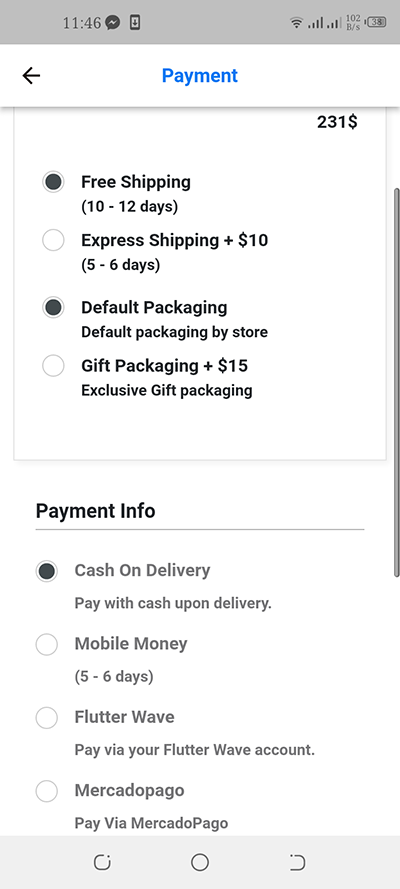This screenshot of a smartphone displays a payment and shipping options screen. At the top, a gray banner contains the time "11:46" in the upper left-hand corner, accompanied by several small icons to its right. On the far right side, typical smartphone status icons for Wi-Fi, signal strength, and battery level are visible.

Just below the banner, the word "Payment" appears centrally in blue font, with a backward arrow on the left side indicating a way to return to the previous screen. This section likely signifies the current step in the transaction process.

The main part of the screen displays various shipping options under the heading. The selectable choices include "Free Shipping (10-12 days)," "Express Shipping (+$10, 5-6 days)," with both options offering "Default Packaging" from the store or "Gift Packaging (+$15)." The radio buttons next to "Free Shipping" and "Default Packaging" are currently selected.

Below the shipping options, the "Payment Info" section provides four different payment method options: "Cash on Delivery," "Mobile Money," "Flutterwave," and "Mercado Pago." The radio button for "Cash on Delivery" is currently selected.

Overall, the screen effectively outlines the user's ongoing transaction steps, displaying selected shipping and payment options clearly.